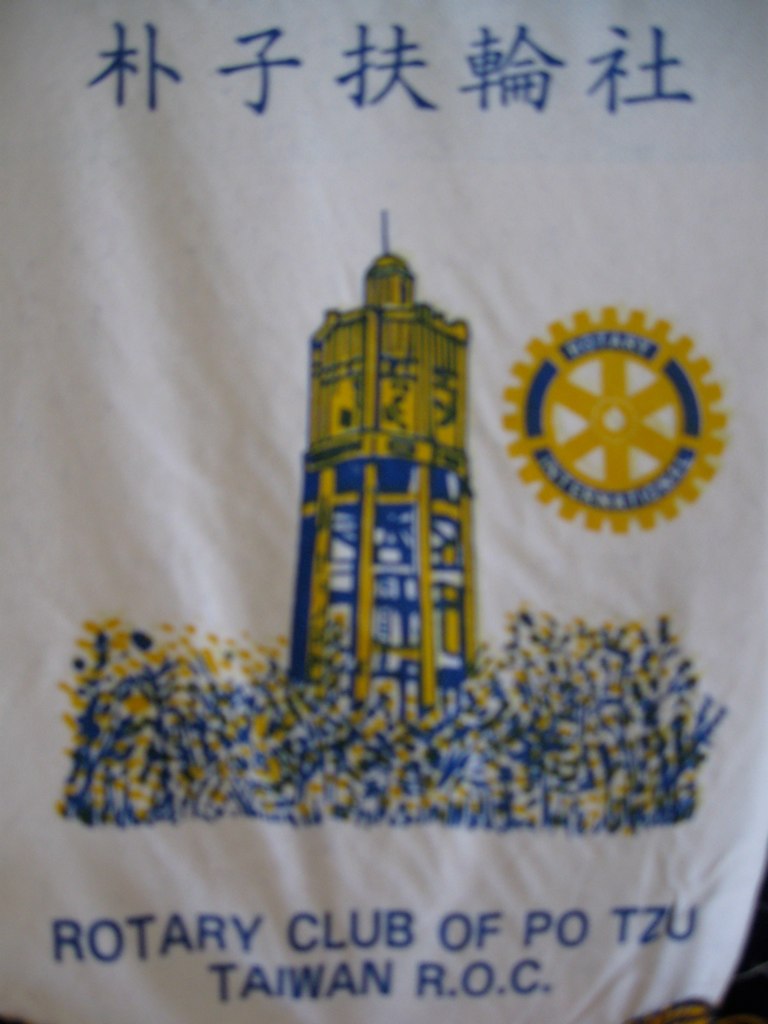The image features a white cloth flag representing the Rotary Club of Taiwan. Prominently displayed in the center is a navy inscription in Chinese or Taiwanese characters. The flag showcases five distinct symbols against the white background. Central to the design is a stylized yellow tower adorned with blue accents, situated amidst a vibrant field of yellow and blue flowers. This composition is complemented by the iconic Rotary Club emblem: a yellow gear with ‘Rotary International’ inscribed in blue around its inner circumference. At the bottom of the cloth, which may be a bandana or a flag, are two lines of blue text. The first line reads “Rotary Club of Po-Tsu,” while the second line denotes “Taiwan, R.O.C.”